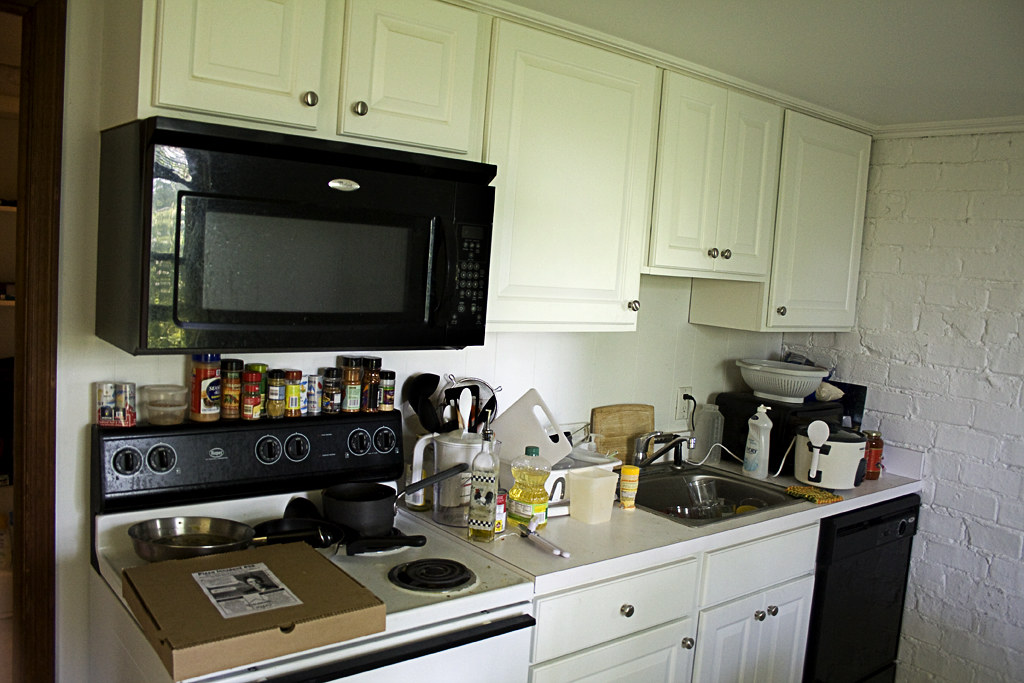This photograph showcases a well-used kitchen with distinct features. The right-hand side wall is adorned with painted white brickwork, presenting a rustic charm. The central section of the image highlights a smooth, white-painted wall, differing in texture from the brick. Above this wall, there are five sets of sleek, white cabinets reaching up to the ceiling. Each cabinet is accented with silver handles, adding a modern touch. 

Underneath the leftmost set of cabinets, a black microwave is mounted on the wall, blending seamlessly into the space with its sleek design. Directly below the microwave, a white electric stove with black knobs is the focal point. The top back section of the stove, where the knobs reside, is lined with various spice containers, indicating a lively cooking area. The stove itself is occupied with a brown pizza box and a couple of pans, ready for use.

To the right of the stove, a cluster of bottles and kitchen items is set against the counter, emphasizing the kitchen’s practical nature. Further to the right, a sink filled with dishes and assorted appliances attests to the kitchen’s active use. This scene captures the essence of a functional, yet cozy cooking space.